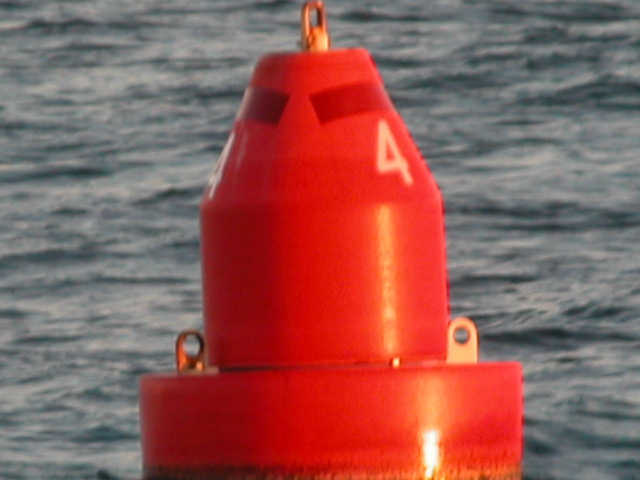This color photograph captures an unfocused buoy floating in bluish-gray, denim-like ocean water, characterized by mild ripples and small white-topped waves. Dominating the foreground, the buoy is a vibrant, bright red, similar to the intense hue of a Crayola crayon, with a distinct cylindrical bottom and conical top that resembles a crayon head. The buoy displays a white number "4" prominently near its upper section. Flanking the rounded base are two golden arched metal pieces with hollow centers, likely chain holes meant for securing or dragging the buoy. Overall, the buoy’s bright red color starkly contrasts with the subtler tones of the restless water beneath the sun.